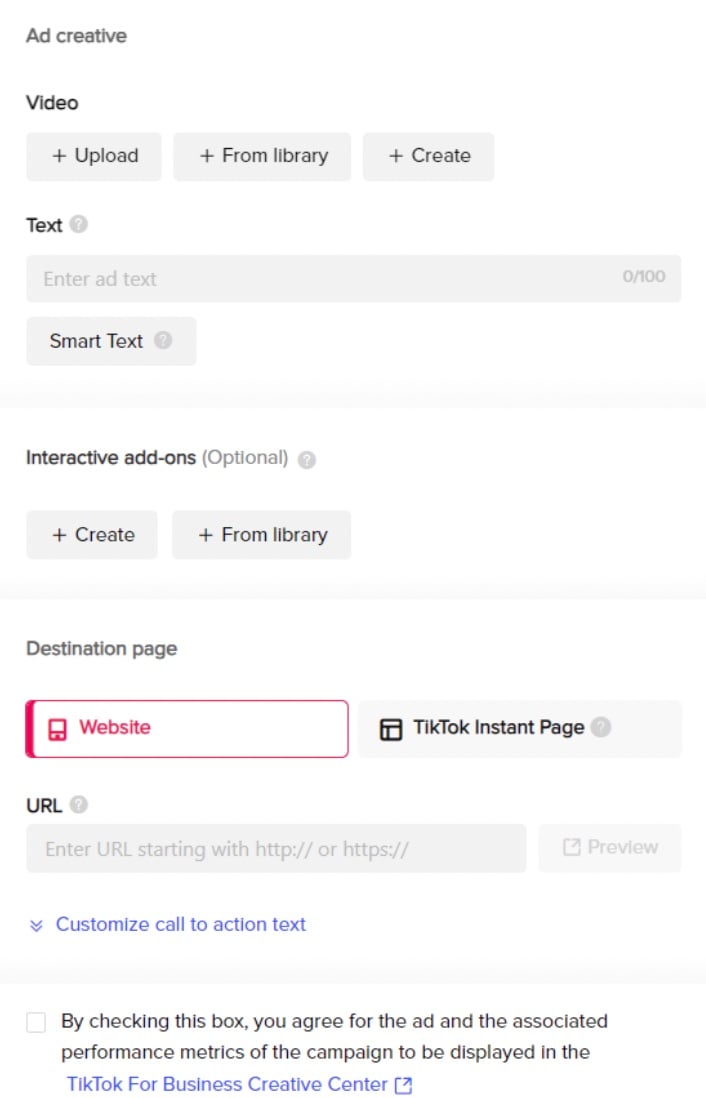The image displays a user interface designed for creating advertisements on a digital platform, primarily focusing on TikTok. The background is mostly white, providing a clean and minimalist look. At the top, the heading reads "Ad Creative." Beneath this heading, there are three prominent buttons labeled: "Upload," "From Library," and "Create," each adorned with a "+" symbol, indicating options to add creative content.

The next section focuses on text input for the ad. It prompts users with "Enter Ad Text" and includes a character count displayed as "0/100," indicating a maximum limit of 100 characters. Below this input field is a gray button that prominently features the text "Smart Text" in black.

Further down, a section labeled "Interactive Add-ons (Optional)" appears, accompanied by two buttons: "Creative" and "From Library," both with "+" symbols. The area designated for the ad's destination follows, starting with "Destination Page." This section allows the user to choose either a website or a TikTok instant page. The "Website" option is styled in red font with a red outline, whereas the "TikTok Instant Page" option is gray with black writing.

Under the destination choices, there's a field for entering a URL, with a prompt to start with "http:// or https://.” A preview button is available in light gray for users to preview their ad.

The final section, highlighted in blue, instructs users to "Customize Call to Action Text." Additionally, there's a checkbox statement indicating that by checking the box, users agree to have their ad and associated performance metrics displayed in the TikTok for Business Creative Center.